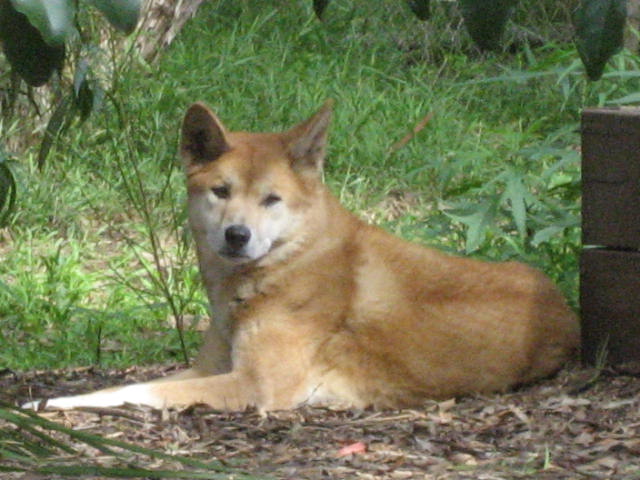In this detailed daytime image, we observe a medium-sized canine, possibly a dog or wolf, featuring a predominantly tan or orangish-brown coat. The animal is lying sideways on a bed of dried leaves or wood chips, with its face turned towards the viewer, revealing a distinctive black nose, small mouth, and very pointy ears. The dog’s face and paws have prominent white markings, extending somewhat into the shoulder and chest area. Surrounding the animal, particularly on the left and behind, is lush greenery comprised of tall grass, shrubbery, and a small tree. Additionally, a brown box is noticeable to the right of the canine. The background suggests a sunlit setting, with sunlight filtering through the leaves, creating a mix of light and shadow, likely indicating a backyard or a natural forestry area.